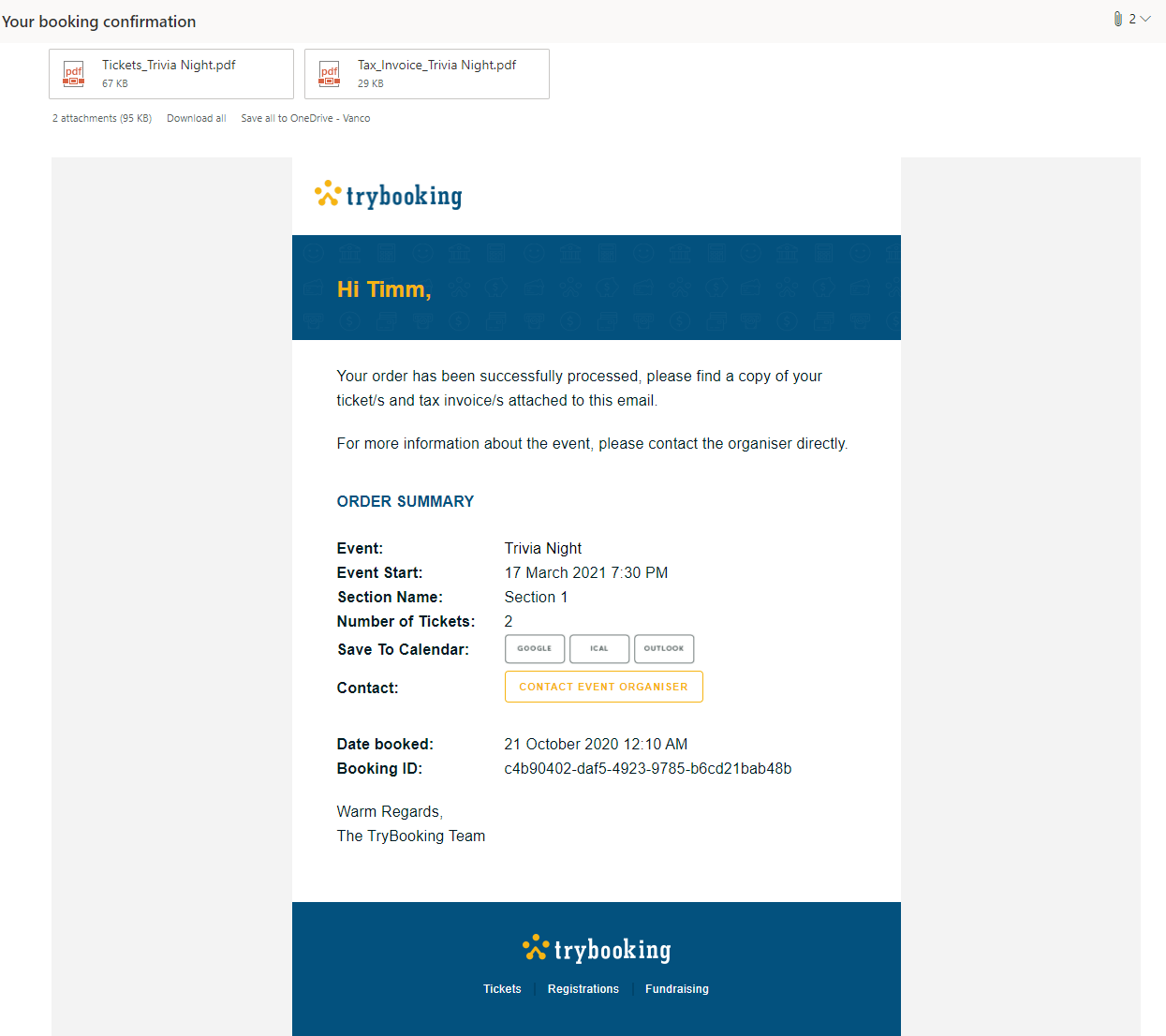In this image, there is a prominent blue box at the top displaying the message "Your Booking Confirmation." Below it, there is a small white box labeled "Tickets" alongside information about a trivia night, followed by another box marked "Tax Invoice - Trivia Night." Adjacent is a section indicating the presence of two attachments.

Further down, a large white box features the title "TryBooking," adorned with a small yellow star shape beside it. Below this, another sizeable blue box greets "Hi, Tim" and includes a message confirming the successful processing of your order, informing you of attached tickets and tax invoices, and advising you to contact the event organizer for more details.

The order summary lists details such as "Event: Trivia Night," "Event Start: 17th March 2021, 7:30 PM," "Section Name: Section One," and "Number of Tickets: 2." There is an option to "Save to Calendar" along with three small blue buttons labeled "Contact." Additionally, there is a yellow button present. Information about the booking date is also provided, stated as "21st October 2020 at 12:10 AM," followed by a unique Booking ID number.

The closing sentiment reads "Warm regards, the TryBooking Team." The image concludes with another large blue box featuring "TryBooking" alongside the same small yellow figure, and headings for "Tickets and Registration" and "Fundraising" displayed beside it.